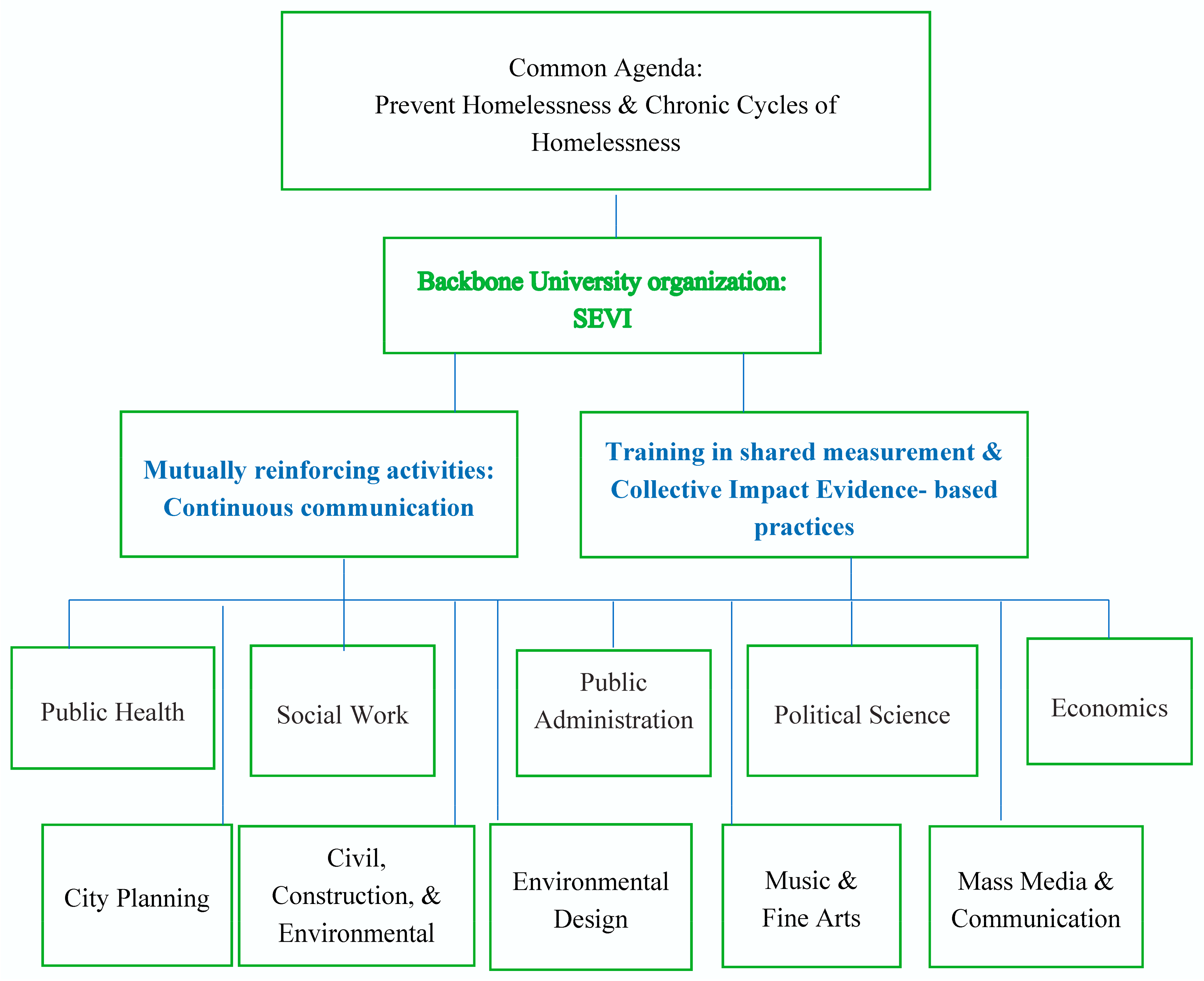The image is a detailed flowchart illustrating the interconnected efforts to prevent homelessness and break the chronic cycles of homelessness. At the top, the chart starts with a box labeled "Common Agenda: Prevent Homelessness and Chronic Cycles of Homelessness." Below this, it connects to the "Backbone University Organization, SEVI." From this central point, the flowchart branches into two major segments: the left box titled "Mutually Reinforcing Activities, Continuous Communication," and the right box labeled "Training in Shared Measurement and Collective Impact Evidence-Based Practices."

Further down, the flowchart expands into a grid of interconnected disciplines, demonstrating a collaborative approach. The left side, from "Mutually Reinforcing Activities, Continuous Communication," leads into "Social Work." On the other side, "Training in Shared Measurement and Collective Impact Evidence-Based Practices" leads into "Political Science."

A broader network emerges from these initial connections, linking various fields: "Public Health," "Public Administration," "Economics," "City Planning," "Civil Construction and Environmental," "Environmental Design," "Music and Fine Arts," and "Mass Media and Communication." These disciplines are interconnected with each other and also align back with the primary activities and evidence-based practices. The interconnected green boxes against a white background visually represent the integrated societal approach aimed at addressing homelessness through varied but linked academic and professional fields.